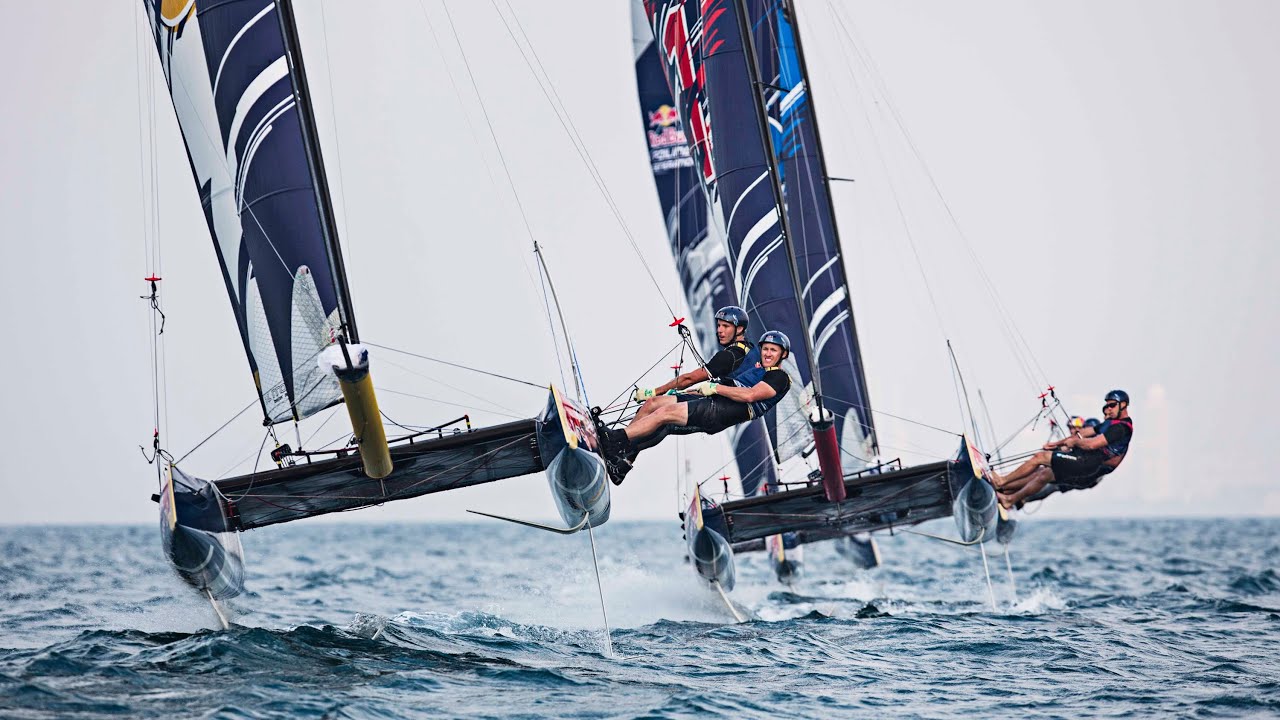This detailed color photograph captures an exhilarating moment in a sailing regatta featuring two high-performance sailboats, each adorned with striking blue and white sails emblazoned with the Red Bull logo. Both vessels, seemingly from the same team judging by the matching blue helmets and black and blue short-sleeved scuba-type outfits worn by the crew members, are lifted dramatically off the water, possibly due to large waves or strong gusts of wind. The boat on the left showcases two crew members, with one man looking ahead intently while the other glances towards the camera with a smile or grimace. Nearby, the second boat appears to be manned by three individuals who are partially obscured but are similarly dressed and equally focused on navigating through the choppy waters. The sailors grip the ropes or cords, hanging off the right side of their respective boats, accentuating the intense action and dynamic movement of the scene. The background features a hazy, cloudy sky with small waves visible at the bottom, adding to the overall drama and energy of the image.